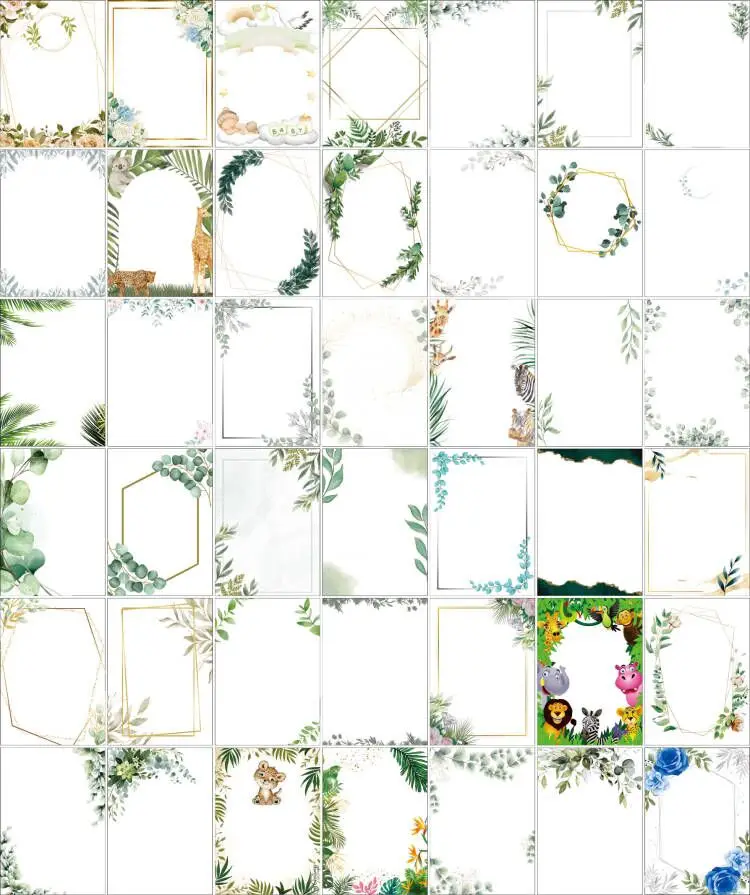The image displays a detailed 7x6 grid of rectangular icons, each showcasing a distinct ornamental border design. Predominantly, these borders feature intricate patterns of leafy ferns in various hues of green, brown, and orange. These designs appear meticulously crafted with some borders presenting elaborate floral arrangements, leaves, and branching patterns. Notably, four of these icons incorporate about 50 charming, cartoonish animals, such as lions, giraffes, koalas, zebras, monkeys, parrots, elephants, hippos, and possibly a lion cub. One striking icon in the bottom right-hand corner features blue roses interspersed with touches of green, outlined by a unique rhombus frame. While many of the borders are characterized by gold and silver curves, some sections of the icons display vibrant, color-rich illustrations amidst sections of white space. The collection evokes a sense of antique letterheads or stationery, possibly intended for personalized notes or craft projects, reflecting a variety of scenarios and tastes.